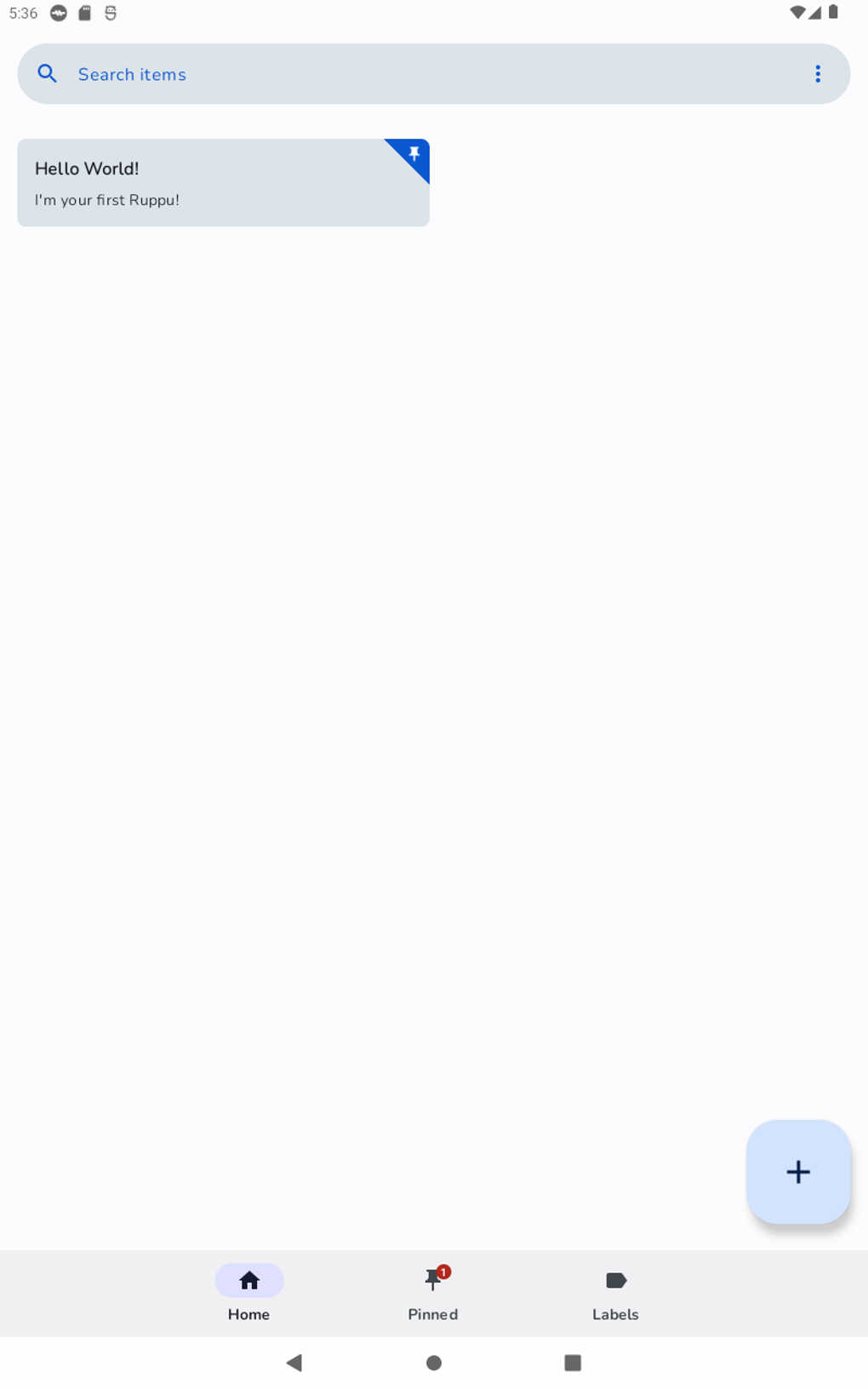This is a detailed screenshot of search results within a mobile application. At the very top, against a light gray background, appears the number "536" in the top-left corner. To the right of this number, there are three icons in succession: a circle icon, an SD card icon, and an "S" icon. Moving further right, in the top-right corner, the status indicators display full Wi-Fi signal, full mobile signal bars, and a fully charged battery.

Directly below, on the same light gray background, is a rounded search bar. The left end of the search bar features a blue magnifying glass icon, followed by the text "Search items" in a matching blue color. On the right end of the search bar, there are three blue dots arranged vertically, indicating additional options.

Below the search bar is a single search result displayed within a light gray rectangle, slightly darker than the background, with rounded corners. The content reads: "Hello World, I'm your first RUPU!" in which "RUPU" is capitalized, and ends with an exclamation mark. Notably, the top-right corner of this rectangle has a blue triangle featuring a white pushpin icon.

The rest of the screen below this result contains substantial negative space until the bottom section, which includes a baby blue square with rounded corners and a black plus sign in the middle, presumably a button.

Further down, a medium gray footer spans the width of the screen, containing three icons. The left icon, a home symbol labeled "Home," is highlighted with a light blue pill-shaped background. In the center is a pushpin icon labeled "Pin," accompanied by a red circle with the number "1" within it, indicating a notification. The rightmost icon is a bookmark symbol, labeled "Labels."

Finally, the bottommost section of the screen features a light gray footer with three navigation symbols: a left-pointing arrow, a circle, and a square, from left to right.